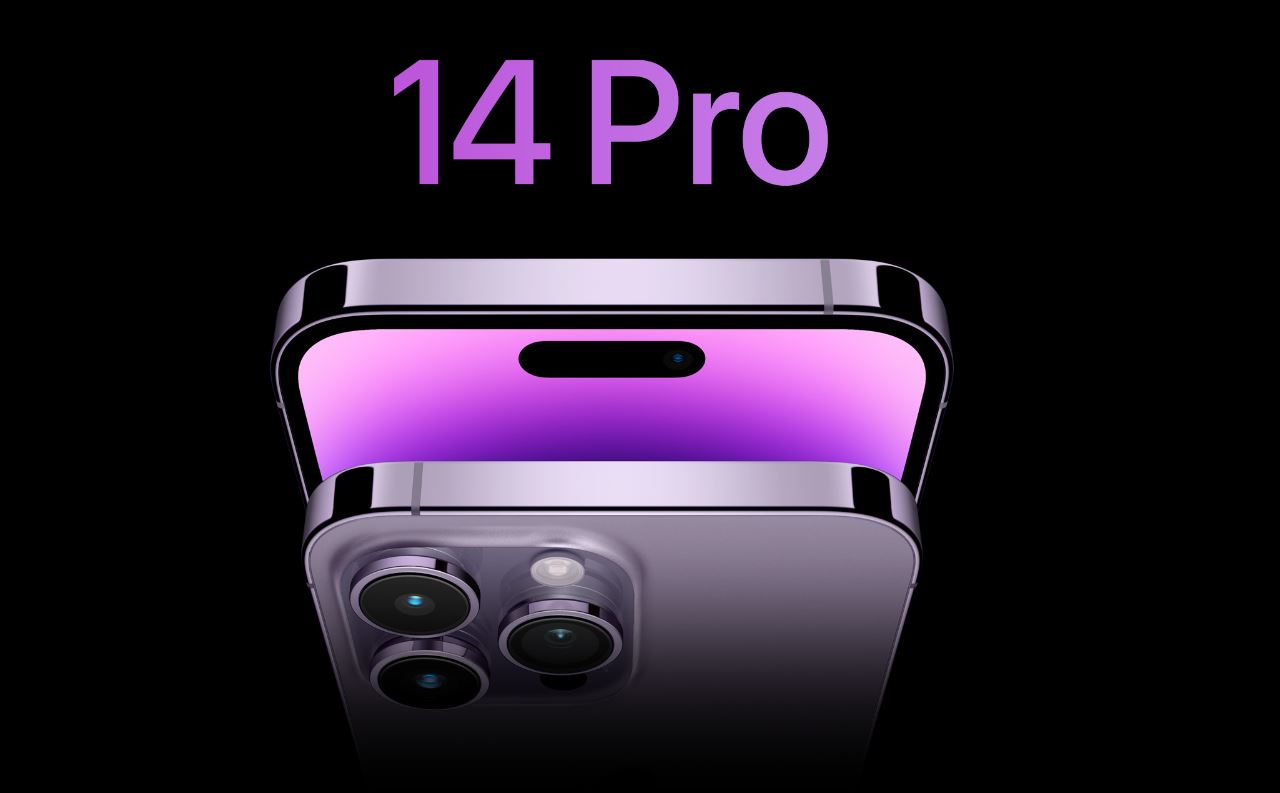This digital advertisement from Apple features a sleek and sophisticated aesthetic with a black background that accentuates the showcased products. Central to the image are two iPhone 14 Pro devices, arranged vertically. The device in the foreground displays the back side, prominently showing off its three lenses and stunning lilac color. Positioned slightly higher in the background, the second device presents the front view, highlighting the sleek design typical of Apple products, complete with a silver edge and minimalistic black outline around the screen. The back panel of this phone appears white or silver, adding a touch of elegance to the overall presentation. The text "14 Pro" is prominently displayed at the top of the image, clearly indicating the model of the phones. This ad effectively combines simplicity and detail, drawing attention to the premium features and design of the iPhone 14 Pro.